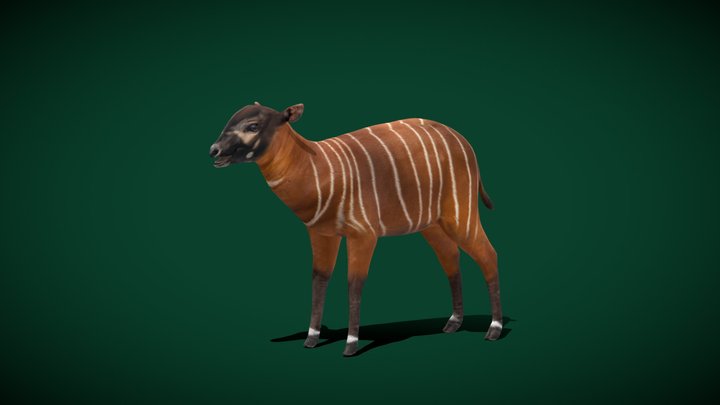The image is a detailed, multi-colored computer-generated piece, horizontally rectangular without a border. The background is a forest-like green, darker in the corners to provide accent. Featured prominently at the center is a four-legged, brown animal with distinct markings. Standing upright, the animal has black hooves encircled by white bands at its ankles. The lower parts of its legs are dark gray, transitioning to light brown at the upper legs and body. Vertical white stripes run thinly from the chest to the hindquarters. It has a black face, short stubby ears, a very black nose, and a small, stubby tail. Sparse white fur accents its eyes. The setting is devoid of text, emphasizing the empty, green backdrop reminiscent of a forest. The detailed features and colored renderings highlight the animal's unique and intricate design.